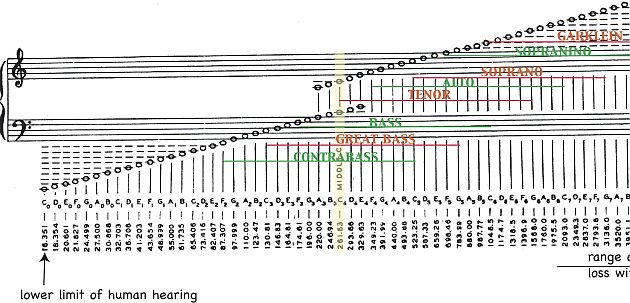The image is a detailed musical chart depicting the range of human hearing, with a focus on various vocal tones. The chart outlines the lower limit of human hearing and includes labels for different vocal ranges such as Contrabass, Great Bass, Bass, Tenor, Alto, and Soprano. The background features horizontal black lines, and the chart is adorned with circles and lines corresponding to different musical notes, which are listed from C to B. Numbers at the bottom indicate specific frequencies, potentially in hertz, starting from around 16.3 and going upwards. The text on the chart is written in multiple colors including black, white, green, red, orange, yellow, and gray. Additionally, the chart includes specific details like decibel levels or frequency limits, aiding in the understanding of the lowest to highest audible sounds for these vocal ranges. The layout features initial text blocks in the bottom left and top right corners, with the vocal ranges centrally placed, extending from the middle to the top right of the chart.